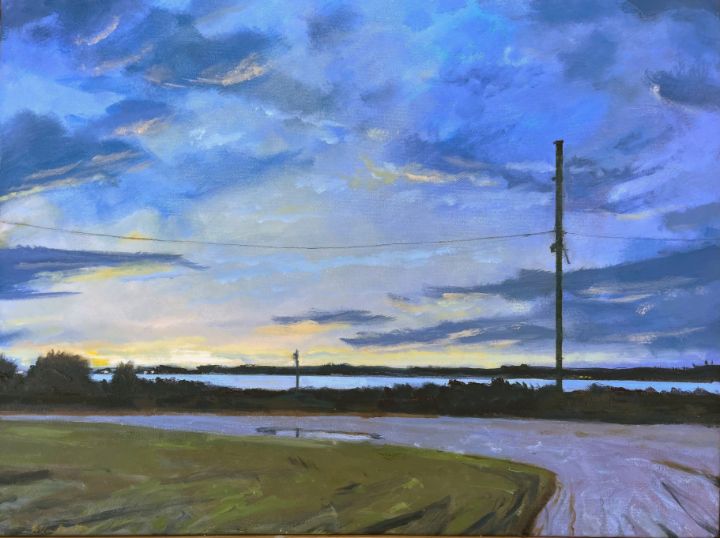This painting depicts an old, muddy dirt road winding from the lower right corner of the image up to the center before curving sharply to the left. The road, brown and filled with rain puddles, is bordered by patches of grass and tall shrubs, whose silhouettes add to the rustic ambiance. A prominent power line pole with wires stretches horizontally across the painting, adding a touch of human presence to the serene landscape. In the foreground, a lush expanse of grass occupies the bottom left corner, contrasting the muddy path. Beyond the road lies a large, calm body of water, possibly a lake, reflecting the tranquility of the scene. The backdrop features a distant line of trees and terrain, with a hint of a small town suggested by tiny, glowing lights. Above it all, the sky is a gradient of blue, purple, and yellow hues, with sun either setting or rising, casting a soft light over the landscape and illuminating dry clouds scattered across the horizon.